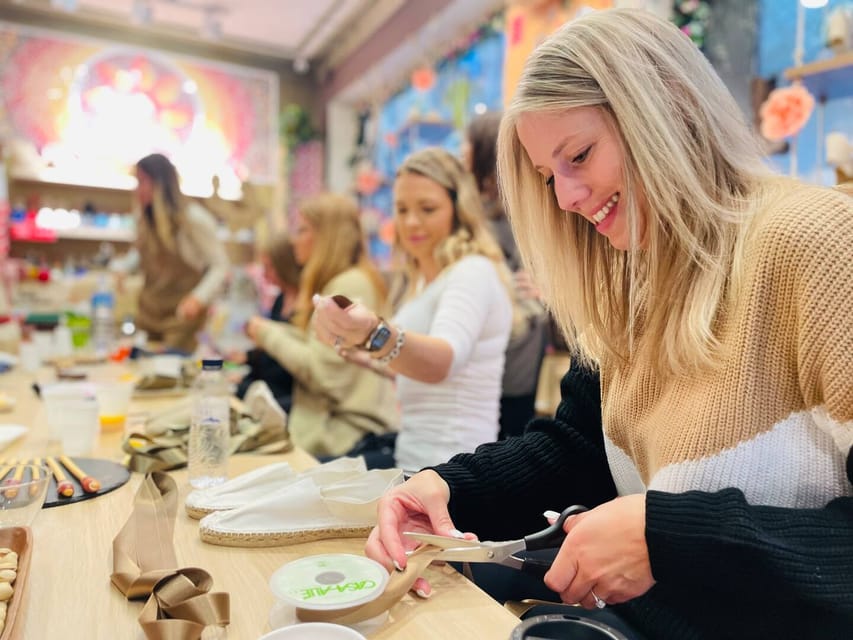In this vibrant and bustling craft store, a woman with medium-length, straight blonde hair sits at a long wooden table surrounded by other ladies, all engaged in a creativity workshop. She's captured in mid-action, holding a pair of scissors in her left hand, cutting a brown ribbon from a spool with a focused but happy expression. Her distinctive sweater features a tan top, white middle, and black sleeves, and she sports a pearl ring on her left hand. The table is strewn with various craft supplies and art materials, indicative of the collaborative and creative atmosphere.

Seated next to her, slightly out of focus, is another participant with medium-length blonde hair. She wears a white quarter-length t-shirt and accessorizes with an Apple Watch and a silver bracelet. In the far background, another blonde-haired lady in a yellow sweatshirt is partially visible, adding to the lively setting.

To the left, a craft store worker with long blonde hair, dressed in a brown apron, stands attentively. The wall behind them glows with a soft pink light, enhancing the bright, pastel-themed ambiance of the workshop. Various bottles and additional craft supplies are also scattered around the table, emphasizing the room's art-centric theme.